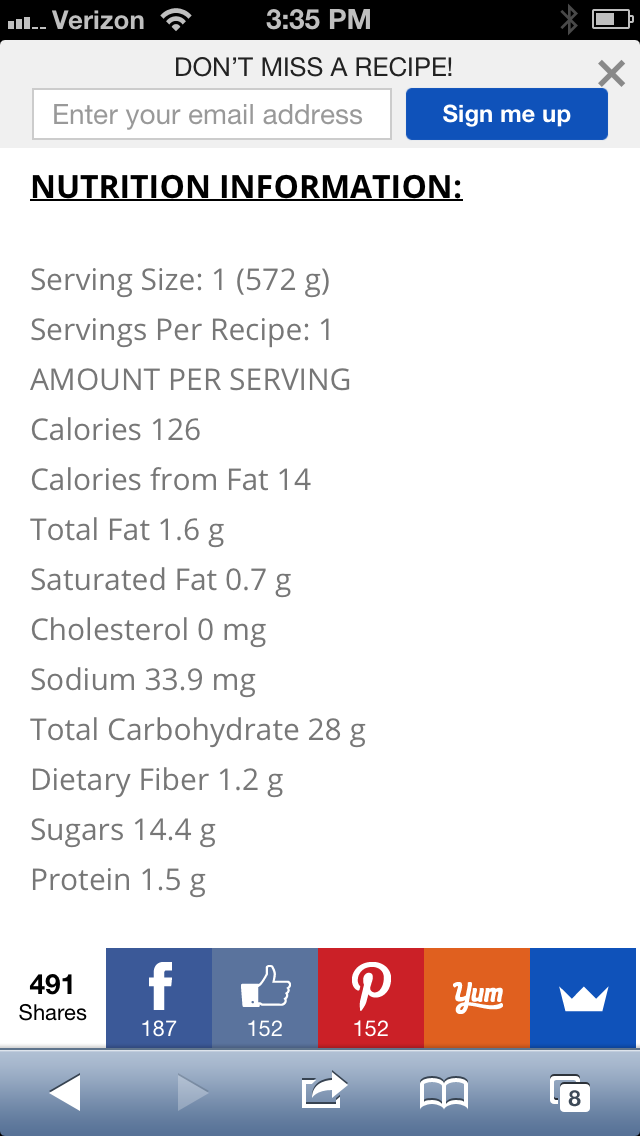The image captures a detailed screenshot on a Verizon phone at 3:35 PM, showing a "Don't Miss a Recipe" prompt. At the top, there are three Wi-Fi bars, the Verizon logo, and a battery icon indicating three-quarters charge. Below that, a gray box urges users to "Enter your email address" and features a "Sign Me Up" button in a blue box. An 'X' is present in the top-left corner to close the prompt. Underneath, bold and underlined text reads "Your Nutrition Information," followed by detailed nutritional values in gray text: serving size (1, 572 grams), 126 calories, 1.6 grams of total fat, 0.7 grams of saturated fat, zero cholesterol, 33.9 milligrams of sodium, 28 grams of carbohydrates, 1.2 grams of dietary fiber, 14.4 grams of sugars, and 1.5 grams of protein. At the bottom, social sharing icons show 491 shares: 187 on Facebook, 152 on Instagram, 152 on Pinterest, an orange Yum button, and a blue button with a white crown. The footer includes navigation symbols: a back arrow, a grayed-out forward arrow, copy, paste, and a book icon, all on a white background with various gray and black text elements.